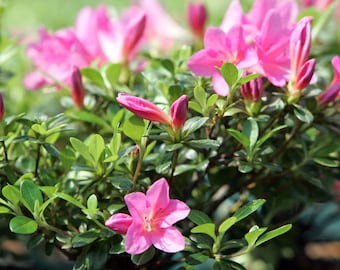This small square image captures a close-up of an azalea plant in full bloom. The foreground is dominated by a singular prominent pink flower situated at the bottom center, showcasing five or six petals with hints of white on the edges and a yellow center. Surrounding it are several green leaves, some of which have not yet opened, indicating that new blooms are imminent. The upper portion of the image is interspersed with additional pink flowers, fully bloomed and in various stages of budding, particularly noticeable in the upper left and right corners. The background is a mix of blurry green foliage and some indistinguishable brown and blue hues at the lower right side, likely part of the outdoors setup that includes a wooden support structure. This detailed snapshot highlights the delicate beauty of the azalea plant against its lush green surroundings, captured in the soft daylight.